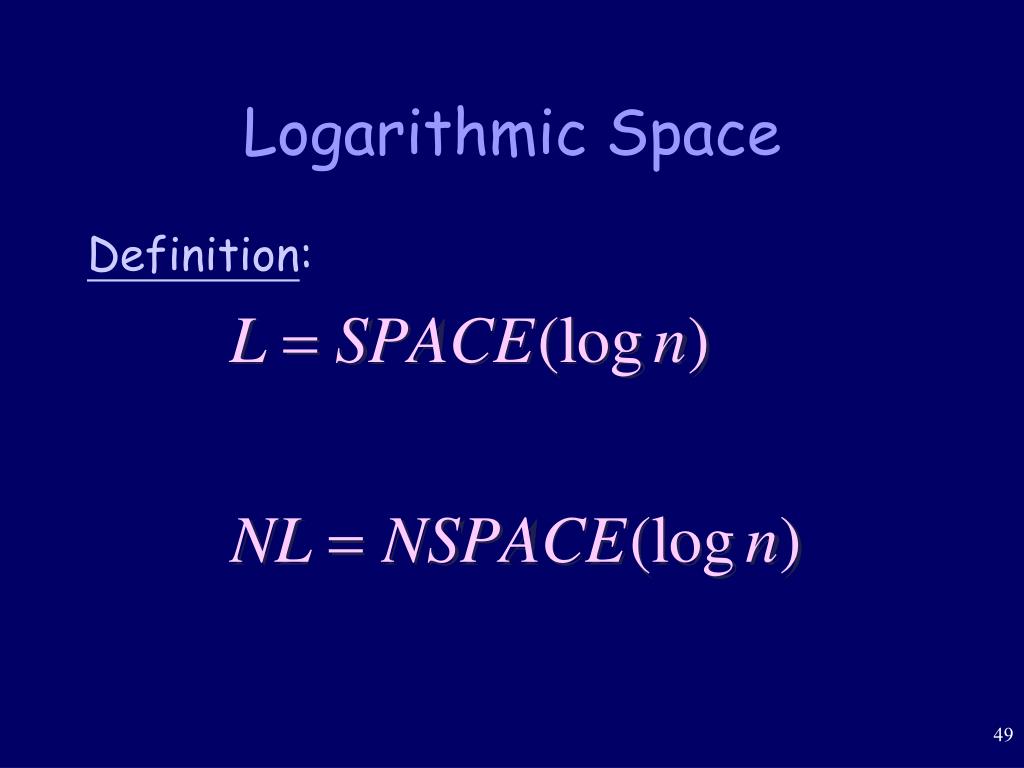The image features a very dark blue square background with the title "Logarithmic Space" printed in a light, light purple, using the Comic Sans MS font at the top. Directly below, the word "definition" is underlined with a colon and printed in white. This is followed by equations written in pale pink with a serif font: "L = SPACE[log]" and "NL = NSPACE[log]". The layout positions the definition text more to the left of the page than the rest. Additional empty space is present on the sides and bottom of the image. In the lower right corner, a small number "49" is displayed.